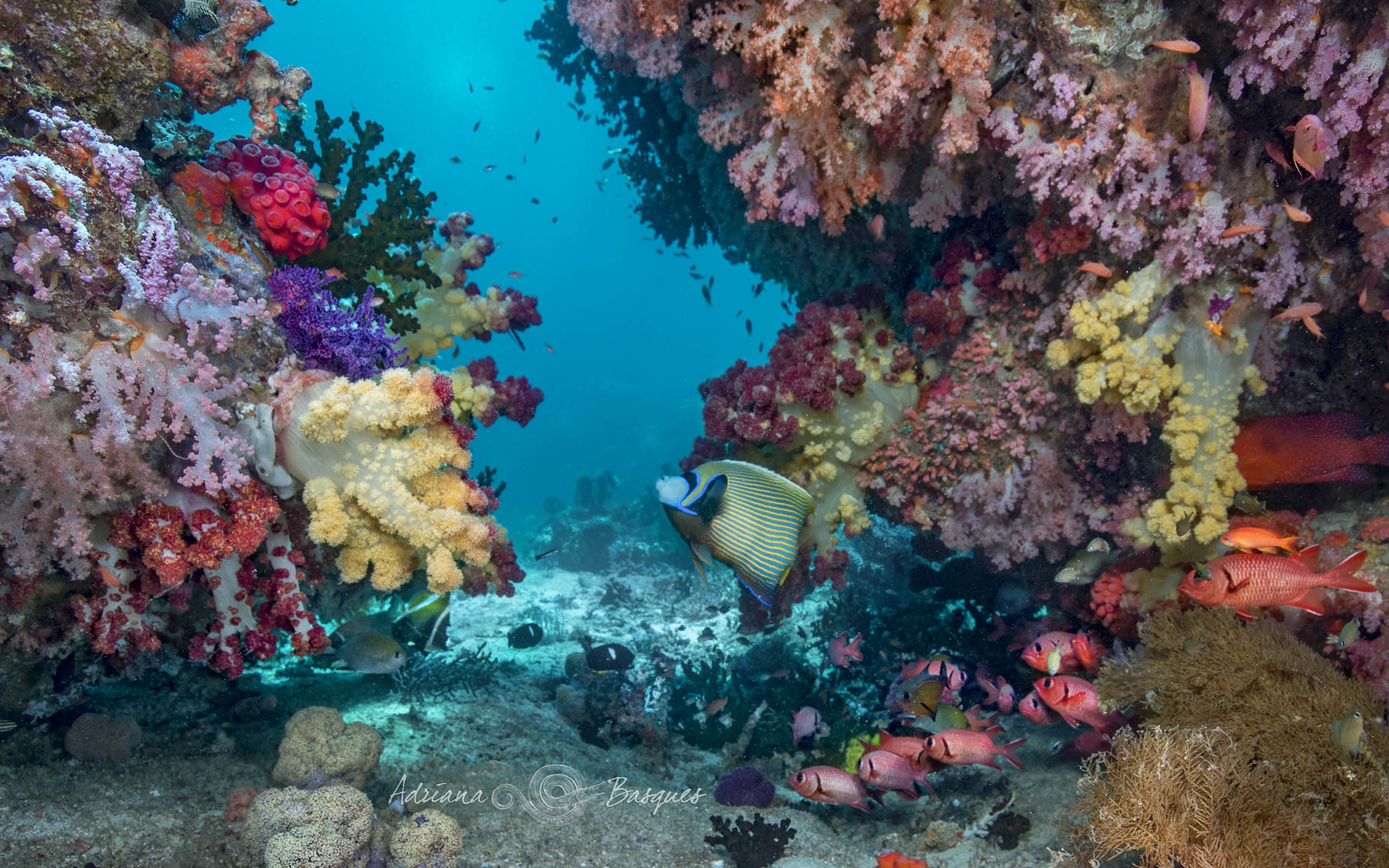In this vibrant underwater photograph by Adriana Vasquez, the image features a breathtaking view of the seafloor teeming with life and color. Central to the composition is a clownfish with striking hues. Surrounding it, a lively school of redfish can be seen near the bottom, while individual redfish and pink fish of varying sizes swim around. The coral reefs on either side exhibit a mesmerizing array of colors, including reds, yellows, oranges, greens, purples, pinks, and darker shades like burgundy. These coral formations create a vibrant frame, through which a diagonal streak of blue sea is visible in the background. Additionally, in the lower center of the image, there is a striking blue, yellow, and white fish, along with black, yellow, and white fish dispersed around the seafloor that is decorated with grainy, gray sand and small coral pieces. Adriana Vasquez’s name is elegantly inscribed at the bottom, completing this colorful and dynamic underwater scene.